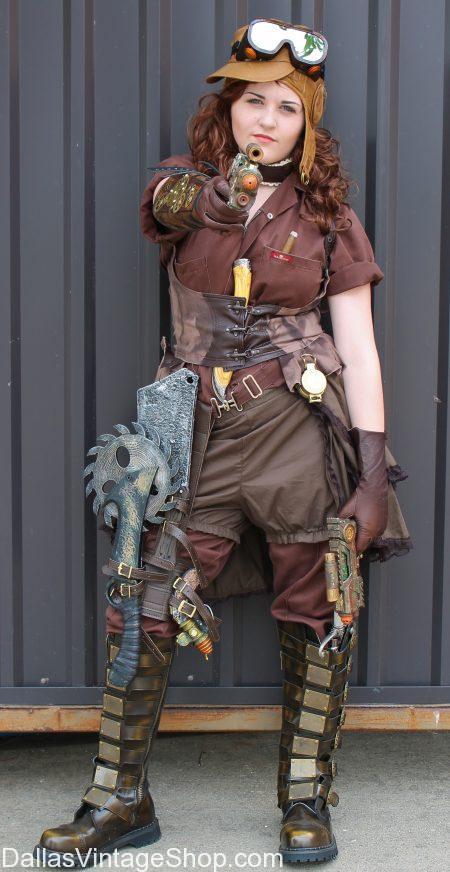In this striking advertisement for DallasVintageShop.com, a young woman embodies the steampunk aesthetic in intricate detail. She stands against a rusted, corrugated metal wall on a concrete floor, her outfit a rich tapestry of maroon, brown, and metallic shades. Her auburn, curly hair peeks out from under a cap adorned with goggles, epitomizing vintage flair. Her ensemble features a rust-colored maroon-brown top and matching shorts, complemented by brown leather boots that are embellished with metal pieces. Straps, holsters, and a buttoned-up vest with old-fashioned styling accentuate her serious demeanor. She wears rust-colored gloves and carries a small, fake gun pointed forward, underlining her readiness for a steampunk or cosplay convention. Additional steampunk elements, including gears, metal, and something resembling a saw blade attached to her legs, complete her elaborate look. With a touch of lipstick and an unwavering, serious expression, she perfectly captures the essence of steampunk in this captivating photograph.